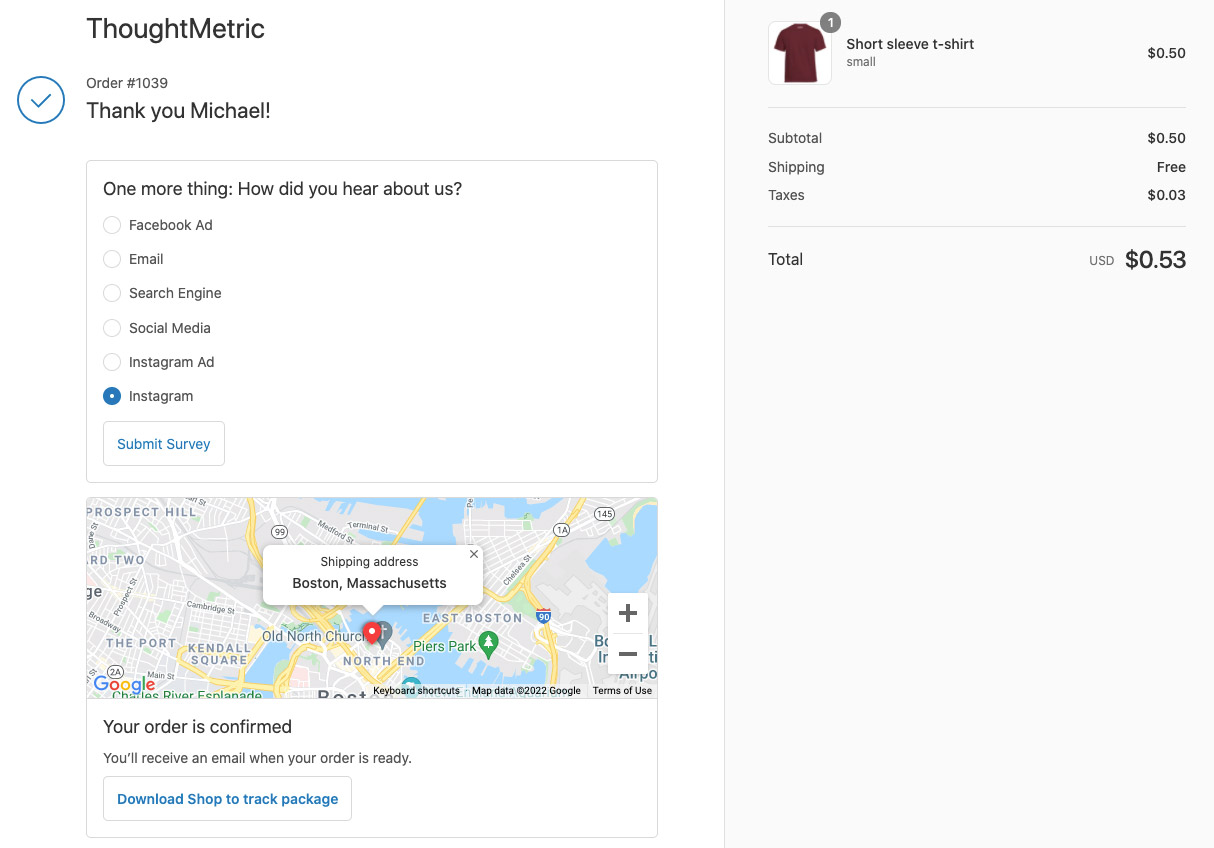In the image, the top left corner features the text "Thought Metric." Below this, there's the order number "1039" followed by a message that reads, "Thank you, Michael!" with an exclamation point. Next, a prompt appears, asking, "How did you hear about us?" with a blue circle beside the word "Instagram." There's a button that says "Submit Survey."

Below this section, a Google Maps display is visible, showing blue for the water and yellow for the streets. In the center, the shipping address is listed as "Boston, Massachusetts," with a red dot marking "Old North Church." Accompanying text states, "Your order is confirmed. You'll receive an email when your order is ready." Below this notification, blue text prompts the user to "Download Shop to Track Package."

On the right side of the image, there's a picture of a burgundy t-shirt. Adjacent to the image, the text reads: 
"Short Sleeve T-Shirt
$0.50
Subtotal: $0.50
Shipping: Free
Taxes: $0.03"

At the very bottom, in black text, the total is shown with "USD $0.53" positioned about five inches to the right.